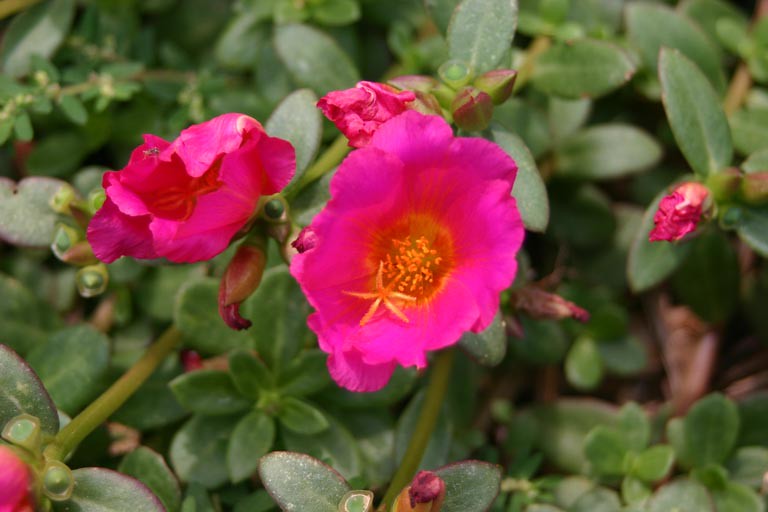This horizontally aligned rectangular image is a close-up shot of a vibrant, fuchsia-colored flower with an orange center, prominently placed at the center. The flower's intricate details, including its tiny seeds, are clearly visible. Surrounding it are green stems adorned with small, oval-shaped leaves. To the left, two additional dark pink flowers can be observed; one is almost fully closed while the other is about half open. On the right side of the image, it becomes somewhat blurry but features what appears to be either a wilting flower or a bud that has not yet bloomed. The corners of the image are slightly out of focus, with the lower left showing a glimpse of another pink flower's bottom part. The background is densely filled with green foliage, making it difficult to see through. The setting appears outdoors, likely in a garden during midday. The harmonious blend of green, pink, yellow, and orange hues suggests a lively natural environment.